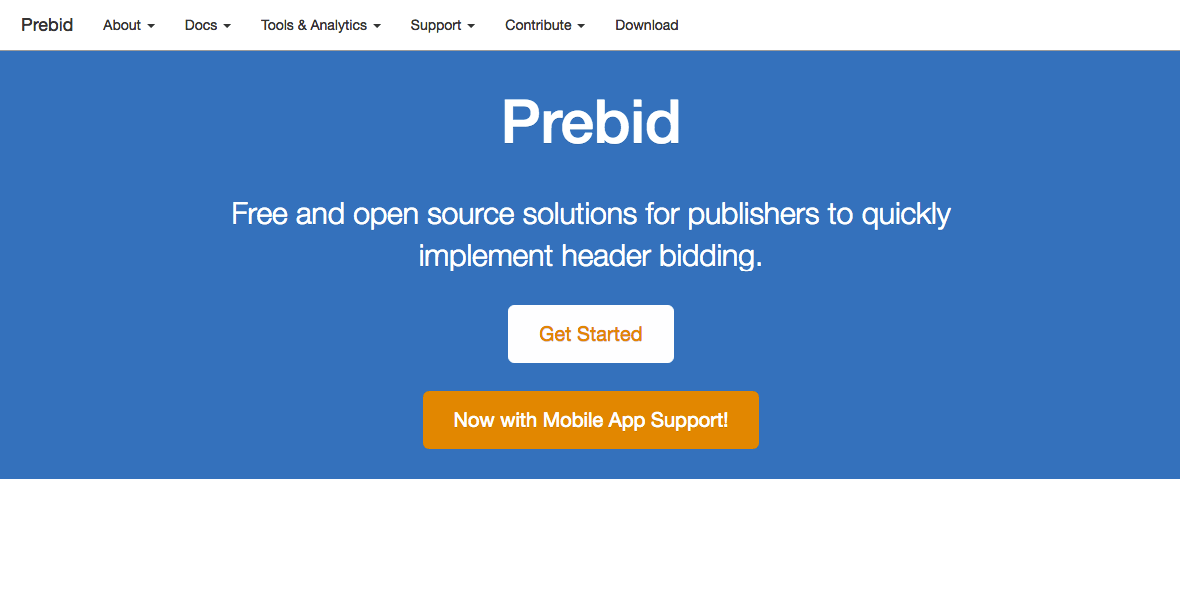The image captures a screenshot of a website titled "Prebid." At the top of the site, there is a navigation bar listing several sections: "About," "Docs," "Tools and Analytics," "Support," "Carterboats," and "Download." 

Prominently featured is a blue rectangle with the text "Prebid" written in large white letters. Beneath this, the tagline reads, "Free and open-source solutions for publishers to quickly implement header bidding." Below the tagline, in a white box with orange text, the phrase "Get Started" is clearly visible, accompanied by a clickable orange button. The button's white text proclaims, "Now with mobile app support!" followed by an exclamation point.

The overall composition of the image features a dominant blue background, with accents of orange, white, and black, providing contrast and drawing attention to key elements.